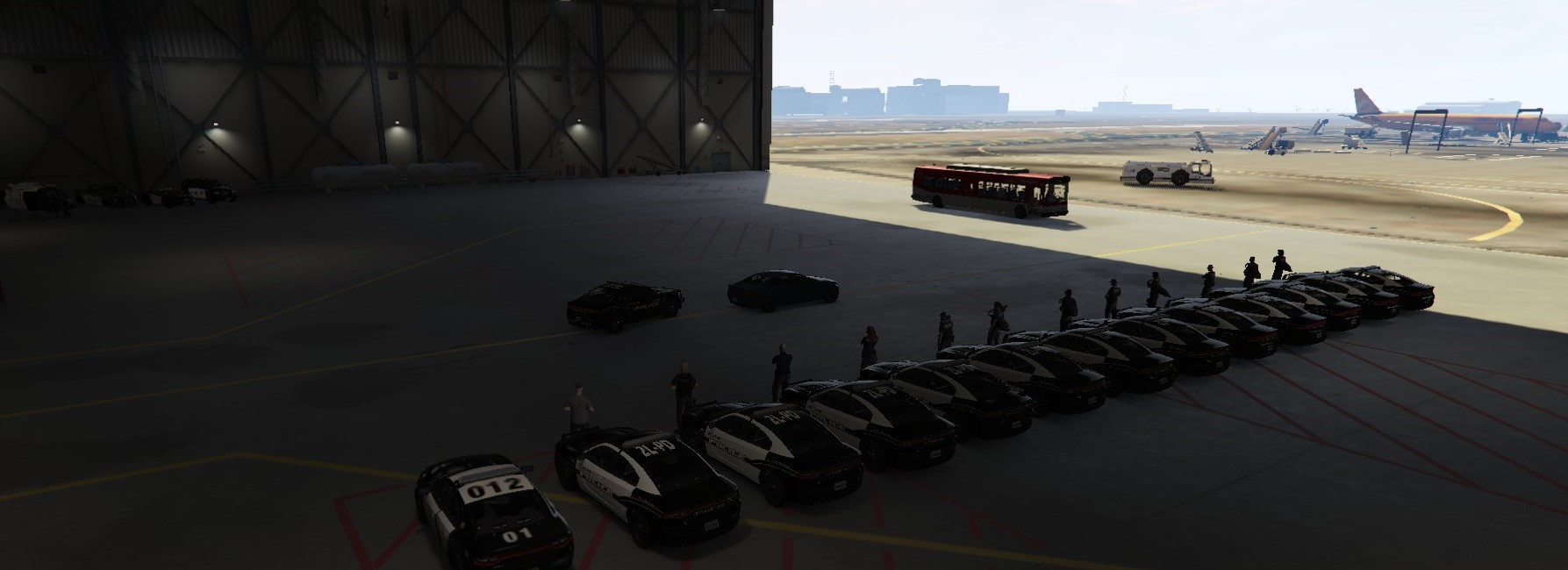The image depicts the interior of a dimly-lit airplane hangar, looking out onto an airfield. Within the hangar, several black and white police cars are neatly parked in a line, each with a police officer standing in front. The hangar is illuminated by some overhead lights attached to dark grey pillars and a grey wall on the left side. Yellow and red markings are visible on the ground, adding to the structured layout of the space. In the distance, beyond the shaded area of the hangar, the bright airfield can be seen. There, an airplane is visible, either parked or moving on the runway, and approaching the hangar is a large red bus. The first police car bears the number "01201," while two of the others display "2LPD." A white truck and a blue car can also be glimpsed in the image, along with additional indistinguishable vehicles and buildings in the distant background, suggesting proximity to an airport. The perspective from high above makes the officers appear small in comparison to the vehicles and vast surroundings.